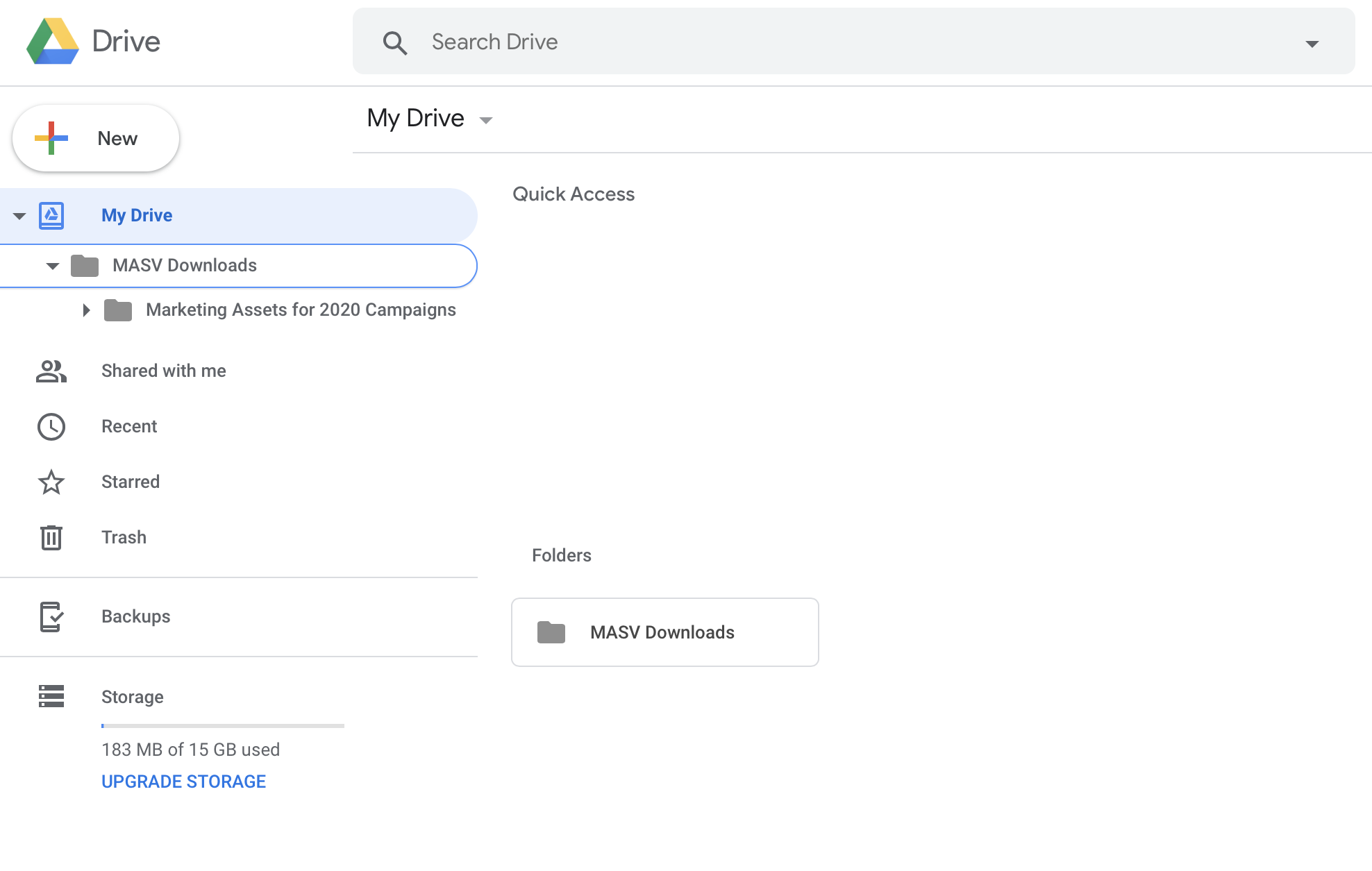A screenshot of a Google Drive interface is displayed. At the top, the Google logo is prominently visible, accompanied by a search bar designed for locating specific files within the drive. Directly beneath the search bar, the "My Drive" section is expanded, indicated by a downward-facing arrow. The only visible content within "My Drive" is the "Quick Access" section, which currently has no visible files.

In the central pane, under the "Folders" heading, there is a single folder labeled "MASV Downloads." 

On the left-hand side, the navigation menu is visible. It includes:
- A "New" button for creating new documents or folders.
- An expanded "My Drive" section showing the "MASV Downloads" folder with a nested subfolder named "Marketing Assets for the 2020 Campaigns."
- A "Shared with Me" section, symbolized by overlapping person icons, indicating files shared by others.
- A "Recent" section, marked by a clock icon, for recently accessed files.
- A "Starred" section, identified by a star icon, for favorited files.
- A "Trash" section, presumably empty as there is no mention of contents.

Additionally, there are sections for backups and storage. The storage indicator shows minimal usage, with only 183 MB utilized out of the available 15 GB. An option to upgrade storage is also present, although it appears unnecessary at this point.